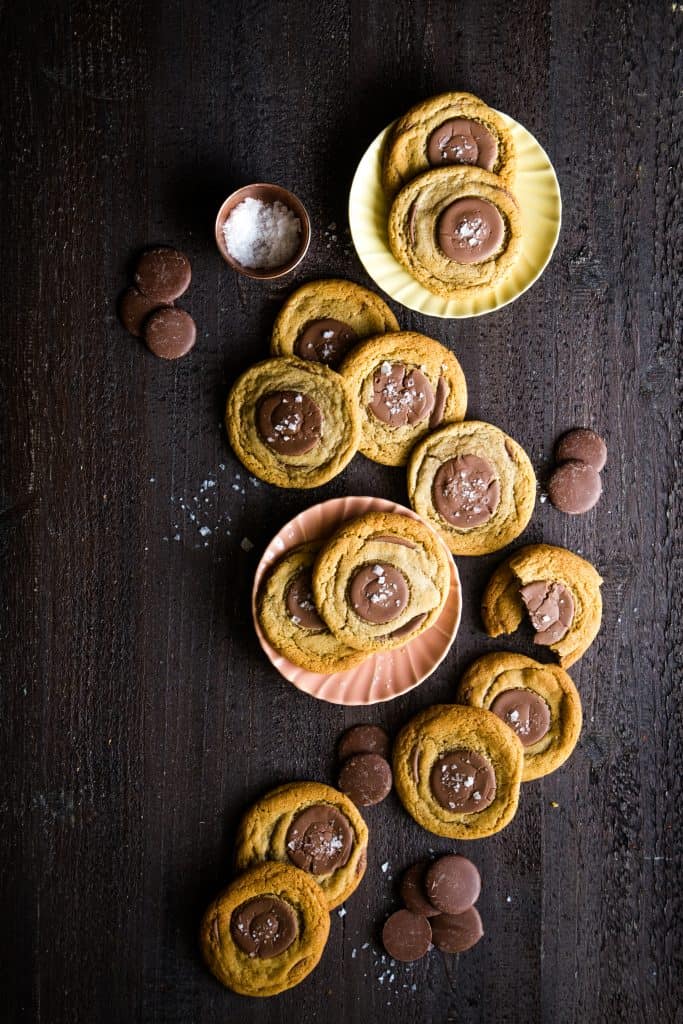In this image, a dark espresso-colored wooden table serves as the elegant backdrop for an artful assembly of circular pastries, resembling cookies. These cookies feature a prominent, round chocolate disc at their center, with a light dusting of what appears to be powdered sugar adding both visual and flavorful accents. The arrangement flows in an aesthetically pleasing, almost S-shaped pattern that integrates both plated and unplated elements. A standout pink plate holds a selection of the cookies, while additional yellow and orange plastic-like plates, with characteristic wavy edges extending to the center, contribute to the colorful and organized display. Besides the cookies, the composition includes a cup of powdered sugar, with specks artistically scattered across the table, enhancing the rustic, yet sophisticated presentation. Each element is meticulously placed, creating a harmonious and enticing visual feast.